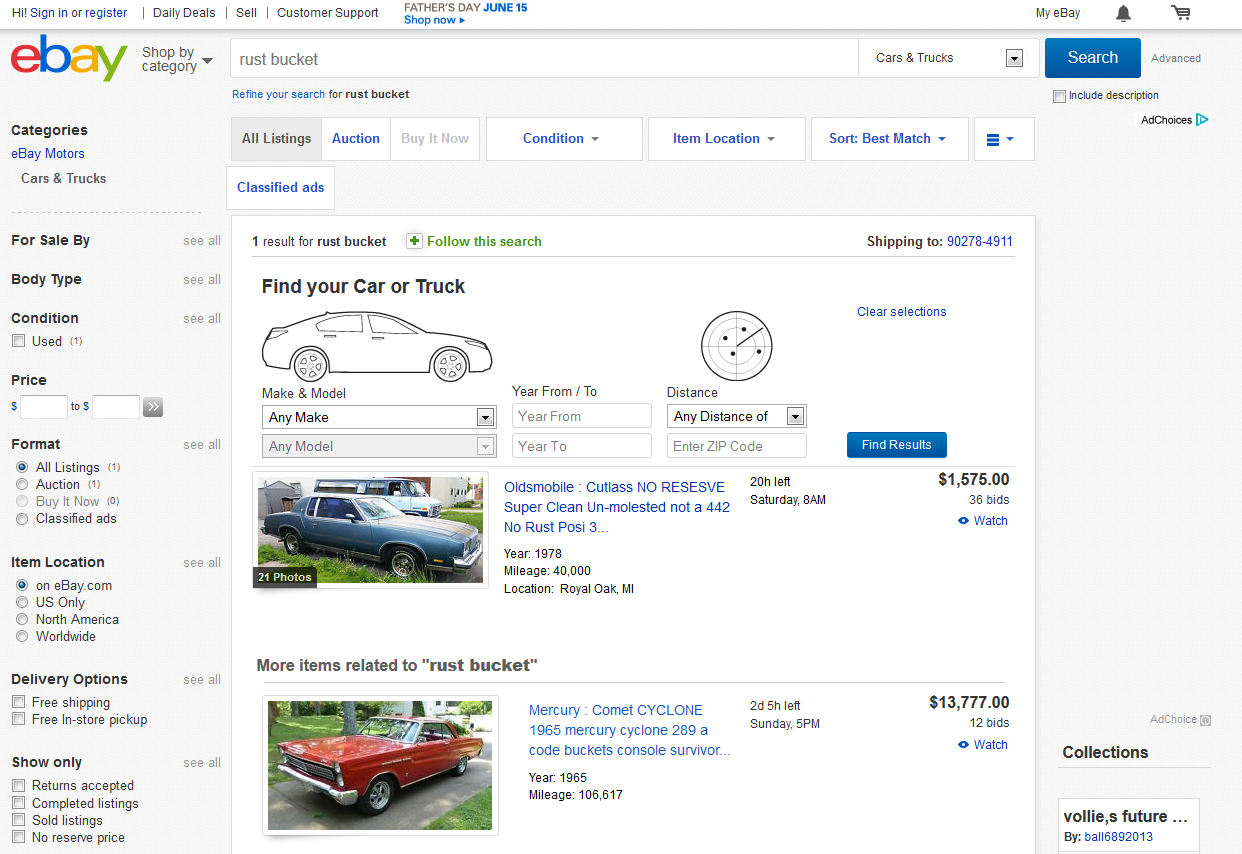This image is a detailed screenshot of an eBay web page featuring a particular search in the Cars & Trucks category. The background of the page is predominantly gray. At the top left corner, the eBay logo is visible along with the "Shop by Category" menu.

A vertical gray sidebar on the left lists multiple categories, including "eBay Motors" and subcategories for "Cars & Trucks." This sidebar also provides filter options for body type, condition (with "used" being selected), and price range input fields. Various listing formats are selectable, including "All Listings," "Auction," "Buy It Now," and "Classified Ads," with "All Listings" currently selected. Filters for item location are set to "on eBay.com" with additional choices for "US Only," "North America," and "Worldwide." The "on eBay.com" location is selected by default. There are delivery options for "Free Shipping" and "Free In-Store Pickup," and show-only options such as "Returns Accepted," "Completed Listings," and "Sold Listings" with "No Reserve Price."

To the right of the sidebar is the main content area, where the user has performed a search for a "rust bucket" within the Cars & Trucks category, selecting "All Listings." The result reveals one listing titled "Oldsmobile Cutlass, No Reserve, Super Clean, Unmolested, Not a 442, No Rust, Pose Three." A blue Oldsmobile Cutlass is displayed beneath this description. Additional search fields below include "Make," "Model" (both set to "Any"), "Year From" and "To," "Distance" with a drop-down menu for various ranges, and an input field for a zip code. These fields are currently grayed out. A blue "Find Results" button is located to the right.

The price for the featured Oldsmobile Cutlass is listed as $1,570, with 36 active bids.